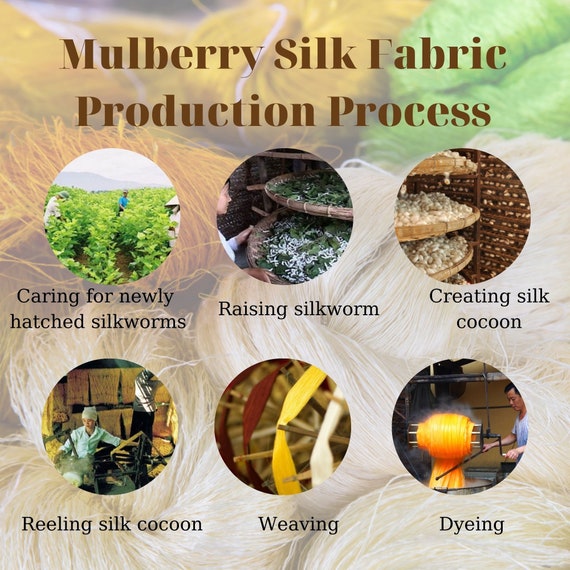This detailed poster, titled "Mulberry Silk Fabric Production Process" in brown letters at the top, illustrates the intricate procedure of producing Mulberry silk fabric against a vibrant background composed of various shades of mulberry silk fibers, transitioning from yellow and green in the upper corners to cream and darker yellow tones around the bottom. The image features six inset circles, each capturing a distinct step in the production process with descriptive captions.

In the top row, from left to right:
1. **Caring for Newly Hatched Silkworms**: This shows a field with mulberry trees and someone working in the background, highlighting the initial care of the newly hatched silkworms.
2. **Raising Silkworms**: A person is depicted tending to trays filled with greenery and silkworms, indicating the nurturing process.
3. **Creating Silk Cocoons**: This circle features several trays now laden with white cocoons, showing the next stage in the lifecycle.

In the bottom row:
4. **Reeling Silk Cocoon**: Illustrates the extraction of silk fibers from the cocoons, with a person operating a reeling machine.
5. **Weaving**: This image shows multicolored silk yarns being interlaced, showcasing the weaving process.
6. **Dyeing**: The final step displays a vivid orange skein of silk being dyed, representing the coloring phase.

The poster not only educates on the comprehensive steps involved in silk production but also provides a visually appealing and informative depiction through its detailed illustrations and vibrant colors.